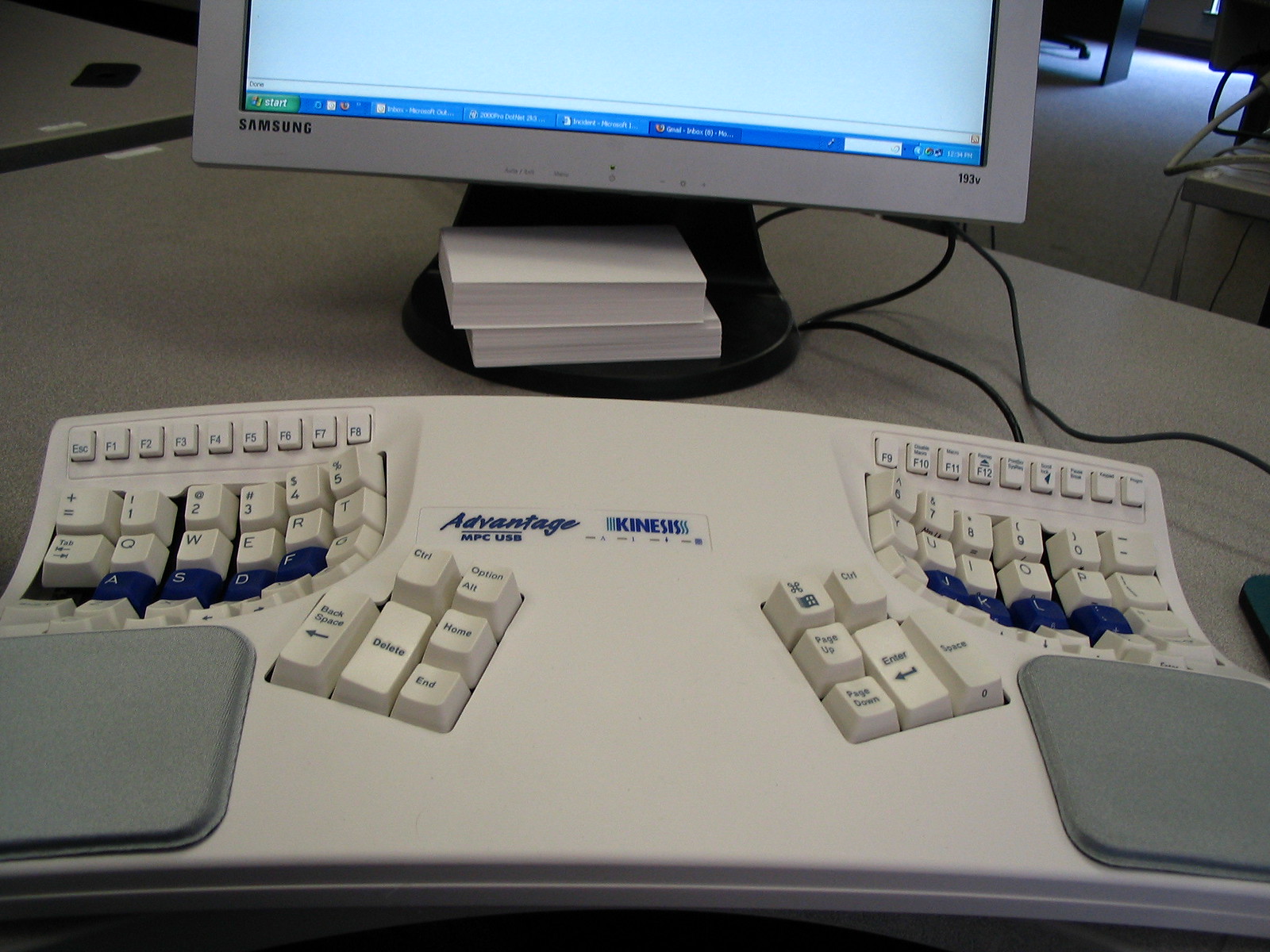This photograph depicts a desktop computer setup in what appears to be an office setting, potentially from the 90s. Dominating the image is an ergonomically designed, split keyboard with the left and right halves of the keys separated and arranged in a curved array to ease wrist strain. The home row keys are colored blue, contrasting with the rest of the beige keys. The left half of the keyboard features eight function keys and the escape key, while the right half contains the remaining keys up to the punctuation marks. Centralized keys such as enter, page up, delete, and home, are situated in the middle section of the keyboard. Two wrist pads, likely made of sponge material, are positioned below each section for additional ergonomic support. The keyboard, labeled with "Advantage MPC USB Kinesis," suggests a model name and manufacturer. Above the keyboard sits a Samsung flat screen monitor with visible cords trailing from the back, typical for older computer models. The setup rests on a white desk, enhancing the vintage office atmosphere.